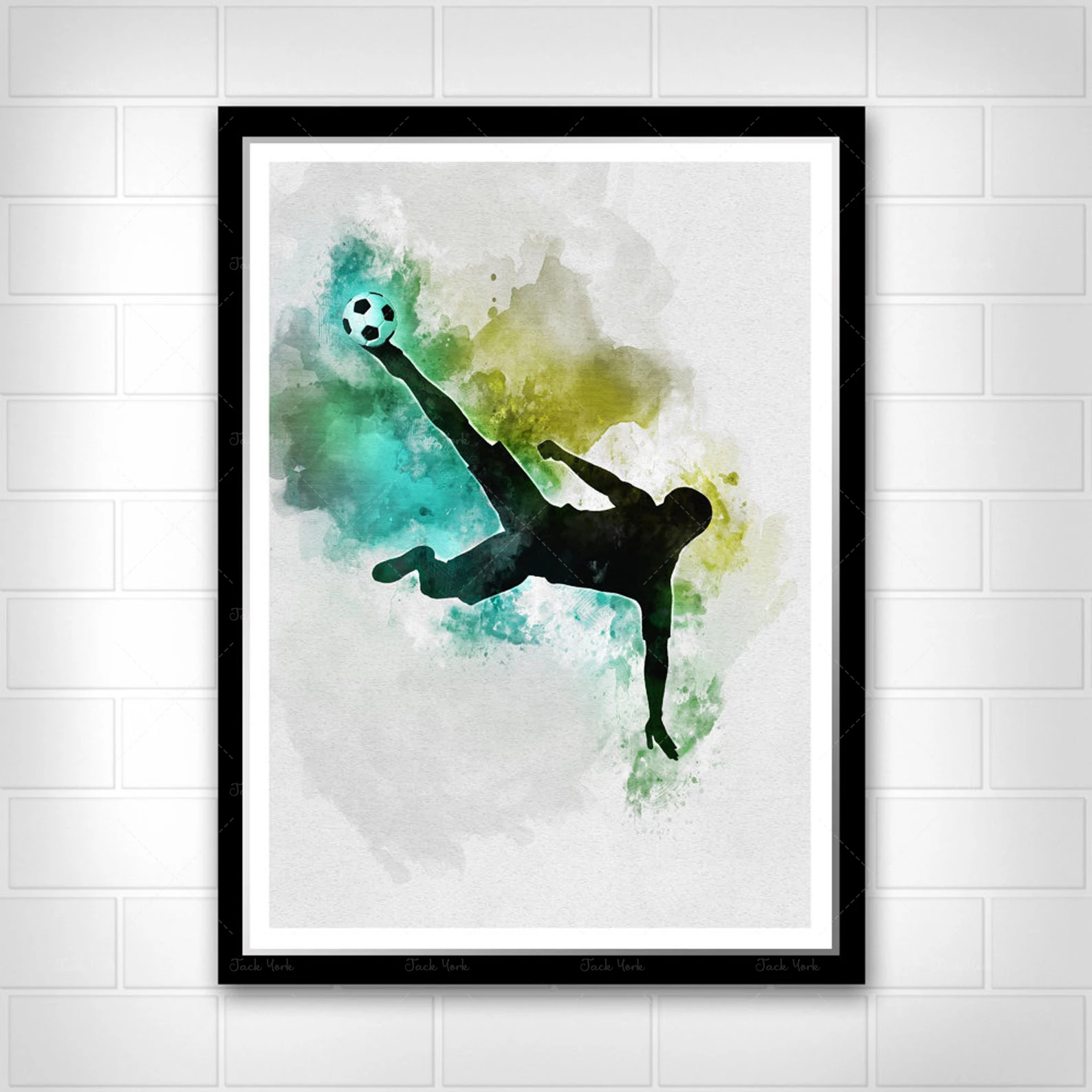The image depicts framed artwork hanging on a white-painted brick wall. The artwork features a black-framed picture with an additional white inner border, showcasing a dynamic silhouette of a soccer player in motion. The player, represented as a solid black outline, is performing an acrobatic bicycle kick with one hand on the ground and his body extended sideways. His toe is in contact with a traditional black-and-white hexagonal soccer ball, positioned in the upper left of the piece, as if he's about to kick it towards a goal. The background of the painting is composed of vibrant watercolor shades including sky blue, turquoise, teal, very light tan, and muted pea green. These colors form abstract blobs that add excitement, action, and contrast to the scene, enhancing the sense of movement and energy captured in the player's pose.